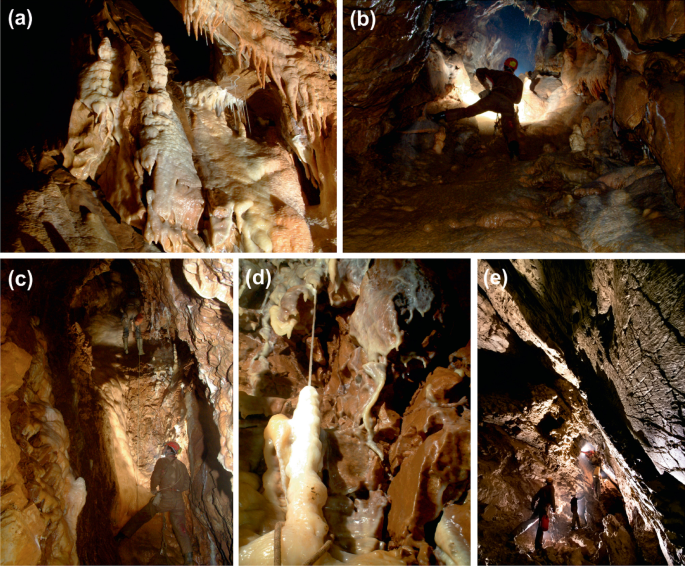The collage consists of five images labeled A, B, C, D, and E, arranged with two pictures on the top row and three on the bottom row. The label text is in white. The images depict the interior of a cave, showcasing a variety of intricate shapes, stalactites, and stalagmites, all in shades of brown and beige. In image B, a man can be seen walking inside the cave. He is silhouetted, wearing a helmet, and holding a flashlight. Image C features another person navigating a tunnel, looking to the left side. The overall setting resembles a detailed cave diagram or photography, capturing the dark, rugged, and rocky environment within.